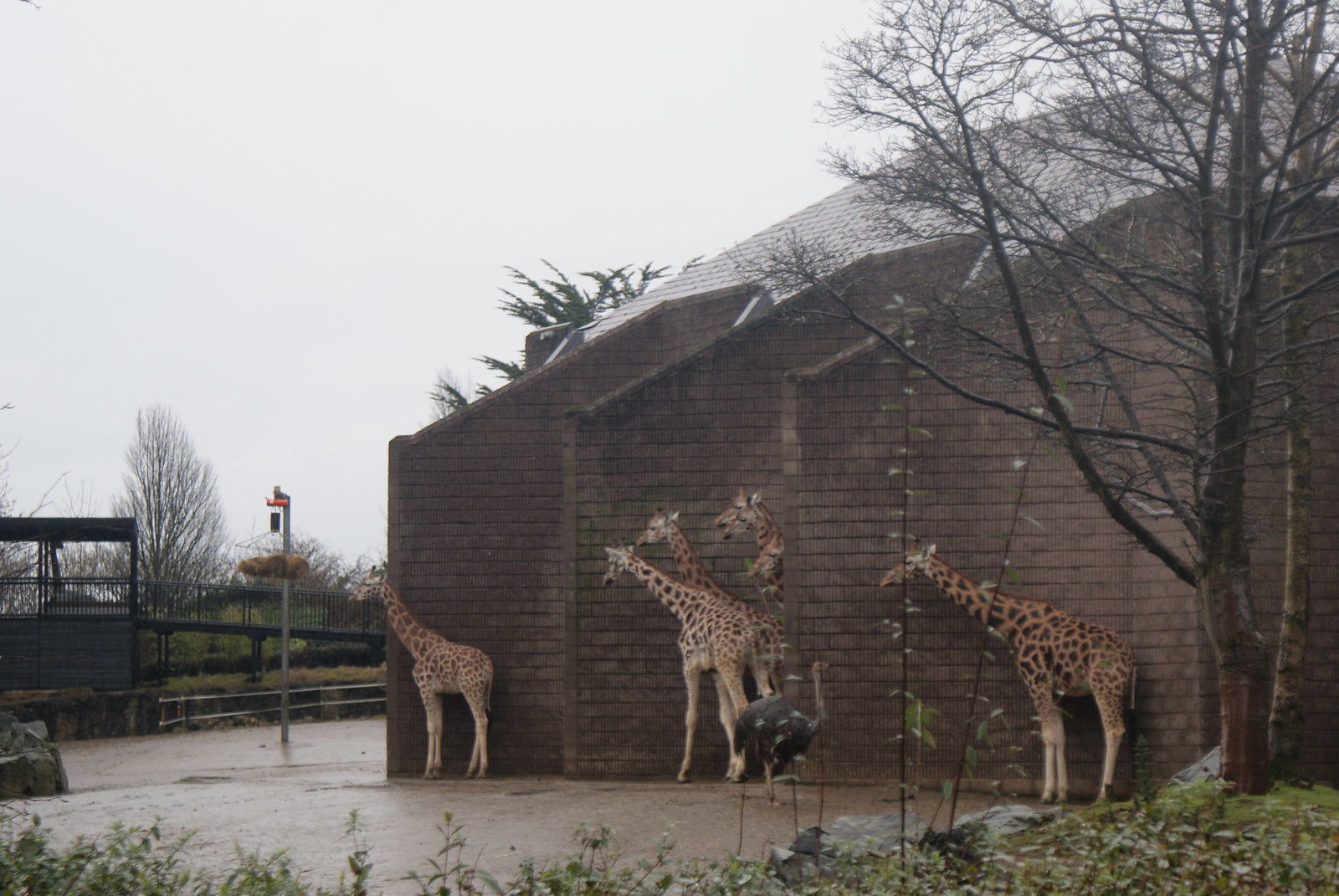This photograph captures a scene of six giraffes and one ostrich within what appears to be a zoo enclosure on a dreary, overcast day. The giraffes, characterized by their brown coats with dark brown spots, are distributed across the enclosure, which features several brick walls with alcoves. The ostrich has a long neck, black body, and long legs, and it stands among the giraffes, staring intently at one of them. The enclosure's ground is shiny and dark brown, possibly wet from rain, adding to the gloomy atmosphere. In the background, there are several tall, sparse trees devoid of leaves, hinting at a winter or early spring setting. Some green grass and bushes appear to be starting to bloom. The sky is filled with gray clouds, suggesting a bleak and rainy day. Each giraffe seems to be seeking some shelter from the inclement weather, with one giraffe standing close against the building's front wall, four gathered between dividers, and another positioned further back. A pole with a light stands near the structure, and beyond the enclosure, there are walkways and possibly a parapet for visitors to observe the animals.